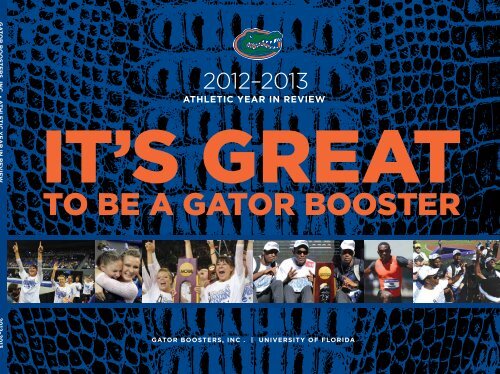The image is a highly detailed cover for the "2012-2013 Athletic Year in Review" for the Florida Gators. The design features a textured background of blue and black alligator skin. At the top, the iconic University of Florida Gators logo—a green alligator head on an orange oval—is prominently displayed. Beneath this, in bold white text, it reads "2012-2013 Athletic Year in Review." Further down, large bold orange text enthusiastically proclaims, "It's Great to Be a Gator Booster."

The central part of the image showcases an array of six photographs capturing various college athletes in moments of celebration and victory. From left to right, the photos depict: two gymnasts with their arms raised in triumph, two gymnasts embracing each other joyfully, a group of women proudly holding an NCAA trophy, three men celebrating behind another NCAA trophy, a sprinter wearing a red and black outfit running towards the camera, and a group of athletes, including a man with sunglasses, jubilantly celebrating.

At the bottom of the cover, in clear white text, it states "Gator Boosters Inc., University of Florida," suggesting that this cover may be used for fundraising purposes or a special publication aimed at supporting the university’s athletic programs.